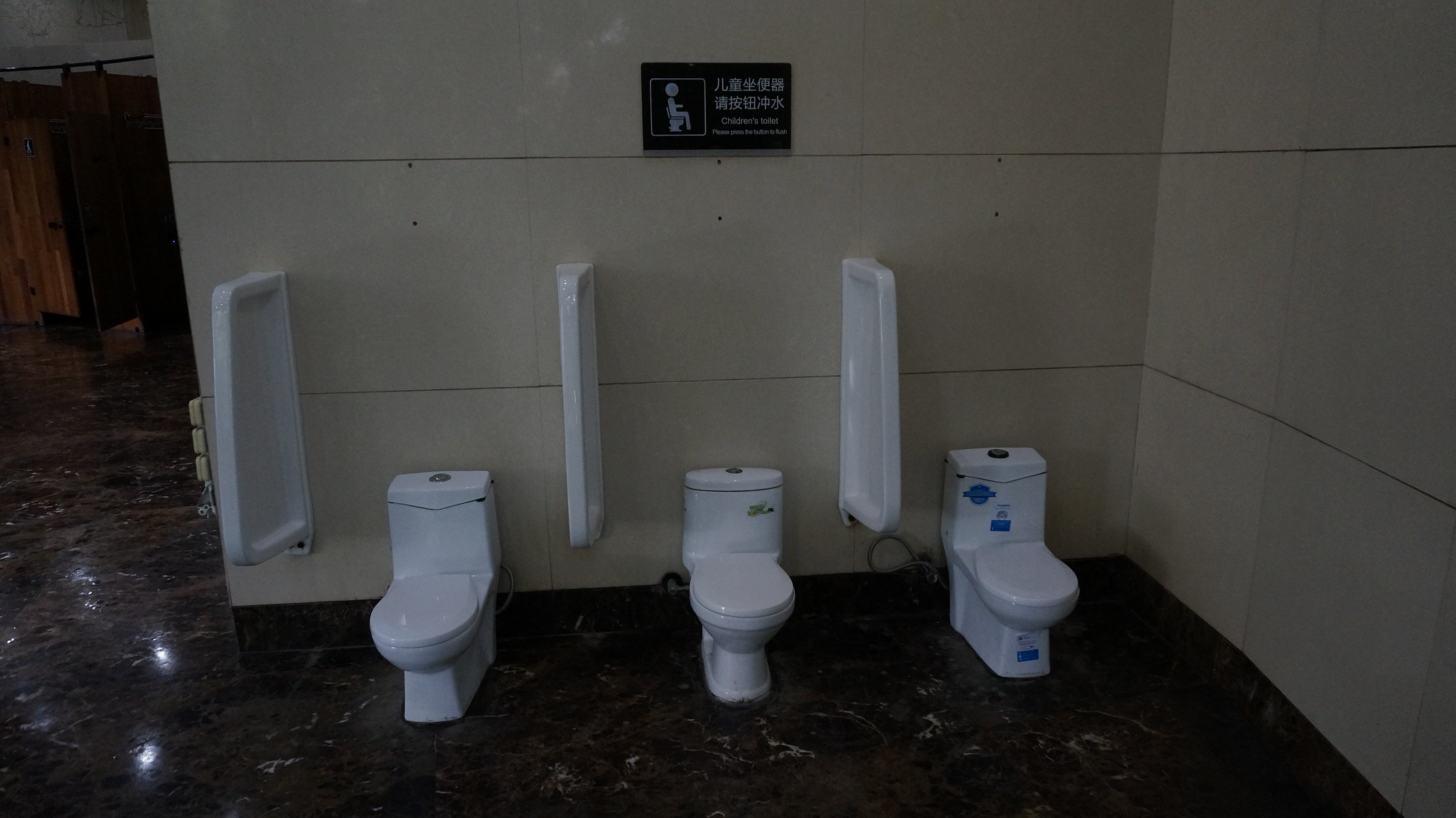This is a photograph of the inside of a bathroom with an open layout, featuring three small, white children's toilets arranged side by side. The toilets are separated by minimal dividers, which extend about a foot and a half from the beige tile wall. These dividers provide little privacy, concealing only the lower parts of the users from a side view. Above the middle toilet, there is a black sign with white text in either Korean or Japanese characters, along with a stick figure visualizing the act of using the toilet. The sign also includes instructions to "Please press the button to flush." The floor is made of black marble with white streaks, contributing a shiny, reflective quality to the space. There is a wide-open area to the left of the toilets, further highlighting the lack of privacy. The walls are tiled with a mix of yellowish and whitish hues, adding to the room's overall light ambiance.